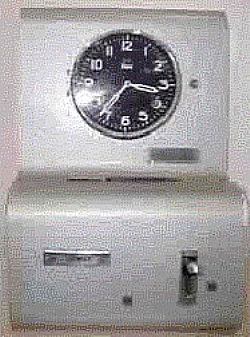The image shows a low-resolution picture of a small, old-fashioned, coin-operated time clock or timer encased in a hard plastic and metal structure. The main focus is the clock itself, which features a black face with white numbers and hands, making it easy to read due to the stark contrast. The clock is rimmed with a chrome or silver border. The top half of the device is slender and flat, painted white, and houses the clock. The lower half protrudes slightly towards the camera and includes two slots – likely for inserting a time card or coin – one located centrally beneath the clock and another slot positioned left to right, probably designed for some other operational functionality. Additionally, there is a silver-colored latch on the front that may operate a mechanism when pushed down. The entire device resembles those found in factories or old coin-operated equipment, and it rests on a brown surface.